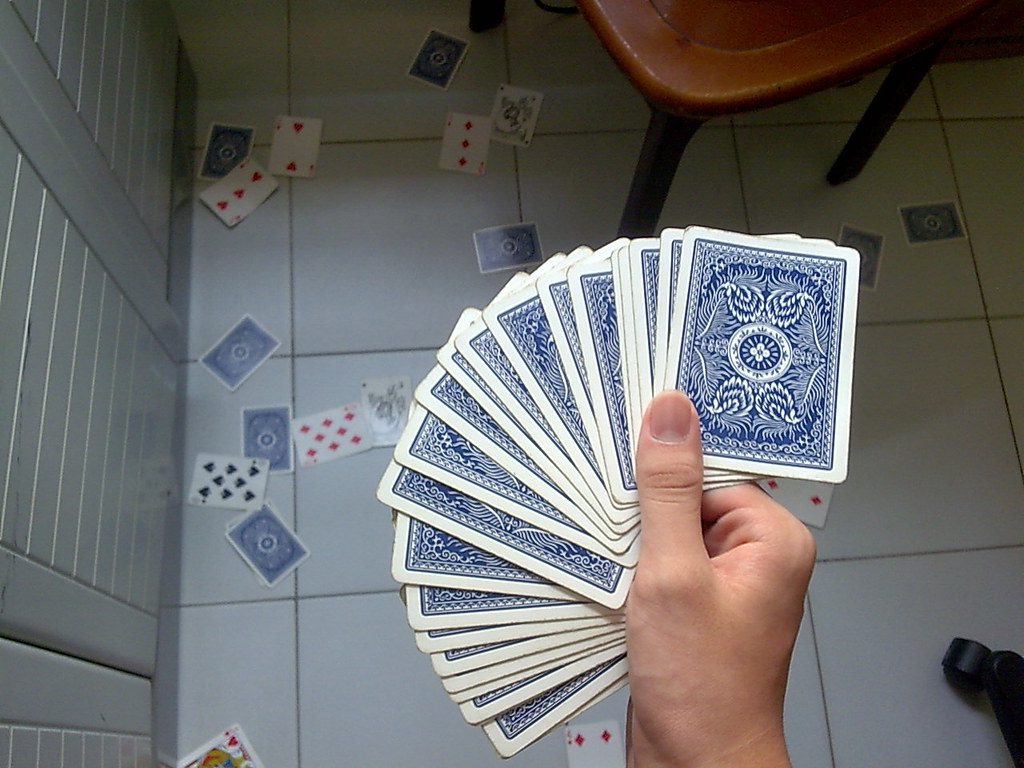A person can be seen holding a deck of cards in their right hand, the cards featuring a blue pattern and positioned face down. The photo is taken from the perspective of the person looking down, suggesting the viewpoint from their head. The white-tiled floor below is scattered with several playing cards, some face up and others face down, reflecting the chaos of a sudden drop. To the left, partially visible folding closet doors blend into the white background, while at the top right, the corner of a reddish-brown chair and a couple of its legs introduce a warmer tone to the scene. Additionally, the bottom right corner features the leg of a black chair with a wheel, anchoring the vignette with its industrial look.